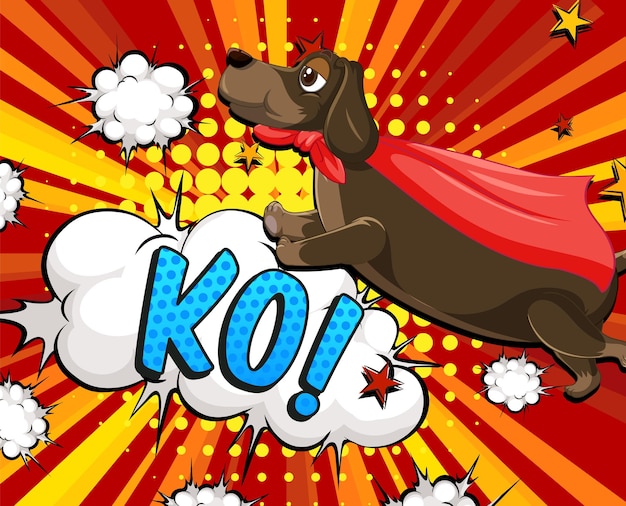In this vibrant cartoonish illustration, a flying brown dachshund with a red superhero cape takes center stage. The dog, depicted in mid-flight with long floppy ears and lighter brown on its muzzle, chest, and feet, strikes an action pose against a dynamic background of red, orange, and yellow rays radiating from behind it. Surrounding the dog are puffs of light and comic book-style stars, contributing to the energetic scene. Prominently featured in the background is a large comic cloud with the letters "KO!" in light blue and darker blue polka dots, complete with an exclamation point and a red star, enhancing the superhero theme. Smaller clouds and stars dot the image, creating a lively and detailed effect reminiscent of a classic comic book.